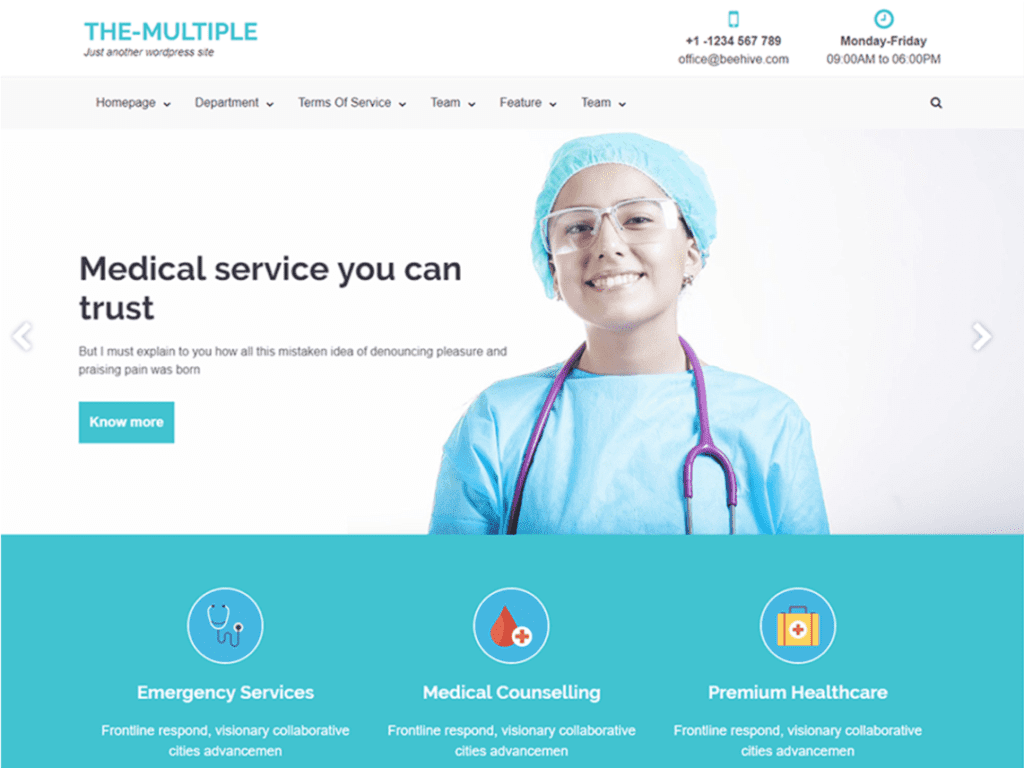Screenshot of a medical company's website showcasing a sleek blue and white color scheme. The top portion of the image features a large, bold header with "THE-MULTIPLE" in capital letters, followed by the tagline "Just another WordPress site." On the right side, the contact information is neatly organized, including a phone number and email address, directly below which the operating hours are displayed with a small clock icon, indicating Monday through Friday, 9 a.m. to 6 p.m.

Dominating the center of the screenshot is a welcoming image of a young woman dressed in blue surgical scrubs. She wears safety glasses and a blue hairnet, and has a purple stethoscope draped around her neck, all while flashing a bright, confident smile. To her left, text reads "Medical services you can trust," followed by an unclear statement about the origins of an idea related to pleasure and pain. Below this text is a blue button labeled "Learn More."

The bottom quarter of the image is taken up by a white banner featuring three distinct icons in a blue strip, each representing different services offered by the company: emergency services, medical counseling, and premium healthcare.